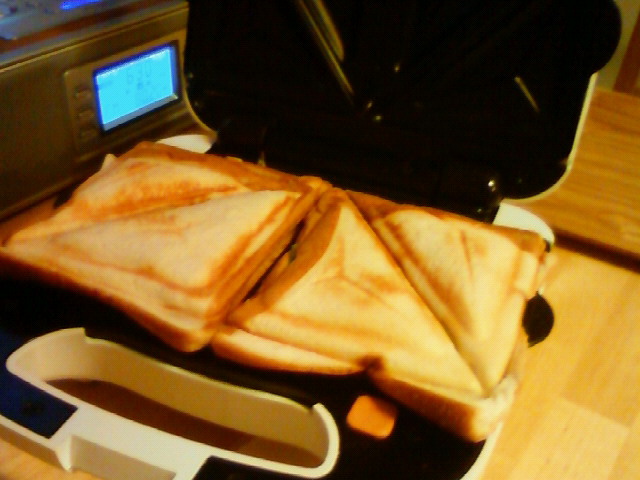This is a high-contrast and somewhat blurry colour photograph of a sandwich press in a kitchen, possibly taken with an AI or a low-quality camera. The sandwich press features a white exterior with black griddles that toast and diagonally cut the sandwiches into triangular halves. Inside the open press, there are two golden-brown toasted sandwiches made of white bread. The sandwiches are divided into four triangular pieces, although it is not clear what the filling is. The press is positioned on a brown wooden countertop, and in the background, on the right side, there is an electronic device, likely a clock radio or possibly a small microwave, with a bright blue digital display. The setting includes a light-colored wooden cabinet door on one side and a metallic object with a blue-lit screen on the other side. Additionally, faintly visible is the outline of a person wearing dark clothing in the background. The overall ambiance of the kitchen includes elements like a wooden table and a light wooden floor, contributing to a homely atmosphere.